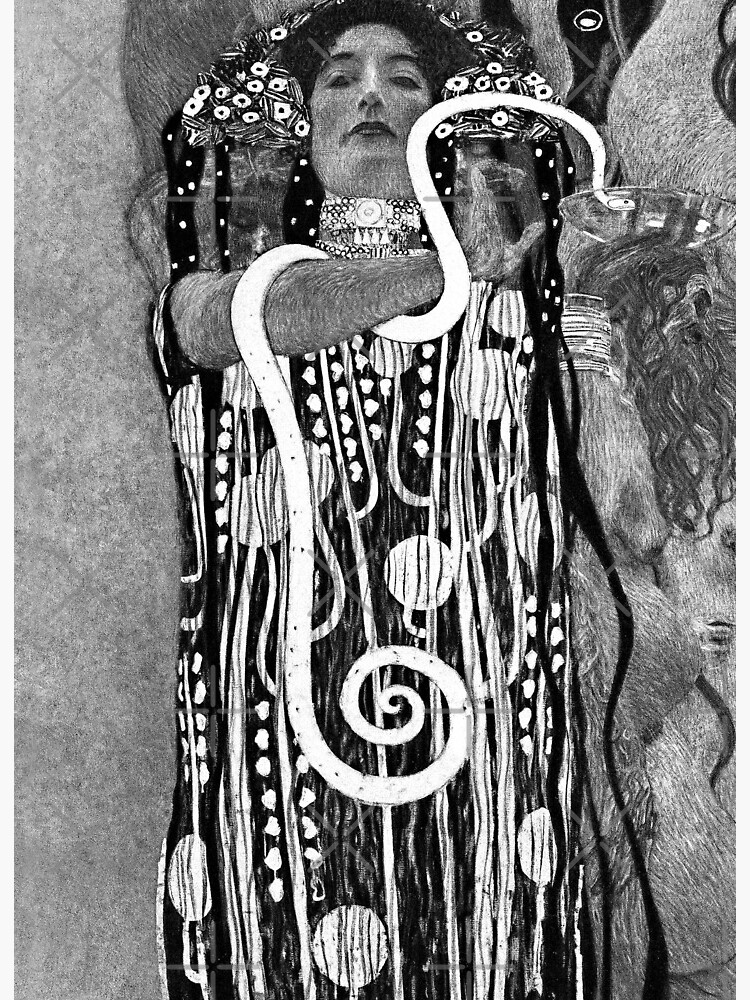This intricate black and white artwork, blending photo realism with artistic rendering, depicts a regal woman adorned in an elaborate headdress and a flowing black garment embellished with white heart-like decorations, vertical lines, swirls, and circles. The woman's long, black hair cascades down past her shoulders, intertwined with the headdress, which is U-shaped and embellished with flowers extending from ear to ear. Her posture is commanding, as she gazes downwards at us from a slightly elevated angle, capturing an air of majesty. Surrounding her neck are multiple chokers, each delicately detailed. She holds her right arm raised and bent at the elbow, with a white snake coiled around it, its head poised slightly above her shoulder and its tail curling down to her midriff. Her left arm supports a plate, upon which the snake's head rests. The background is filled with abstract, rock-like structures and faint animal imagery, contributing to the ethereal and mysterious vibe of the scene. The entire composition, rendered with pencil and charcoal shading, commands attention through its textured depth and intricate detailing.